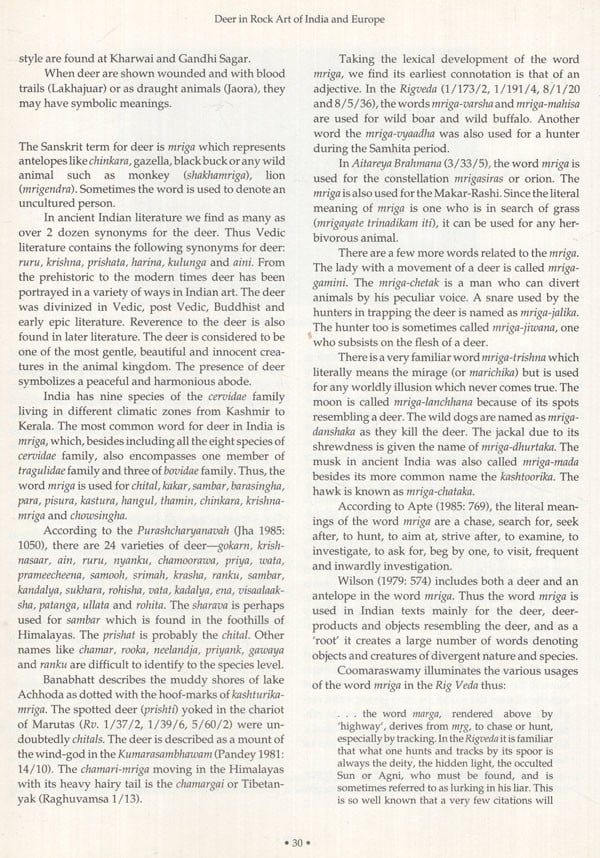This is a scan of an off-white page from a book, featuring black text formatted in two columns with multiple paragraphs per column. The page is headed with the title "Deer in Rock Art of India and Europe." The page number, which appears to be 30, is printed at the bottom with decorative symbols flanking it. The text begins mid-paragraph, continuing from the previous page, discussing the stylistic representations of deer at Karwe and Gandhi Sagar. It mentions that wounded deer with blood trails or those depicted as draught animals may hold symbolic meanings. There is a detailed explanation on the Sanskrit term for deer, "Mriga," which encompasses species such as the chinkara, gazella, black buck, and other wild animals, and can even refer to uncultured individuals.

The text also highlights that ancient Indian literature includes over two dozen synonyms for deer, revealing their cultural significance. Examples from Vedic literature include synonyms like Bruru, Krishna, Prashait, Harina, Kalunga, and Aini. The portrayal of deer spans from prehistoric to modern times in Indian art, characterized by their divinization in Vedic, post-Vedic, Buddhist, and early epic literature. Further down, the text describes the deer as representing a peaceful and harmonious presence, revered across various historical and literary contexts. The narrative concludes with a note referencing Wilson (1979), which discusses the term "Mriga" and its application to both deer and antelope. Despite the slightly out-of-focus quality, this page provides a rich, intricate account of the symbolic and cultural roles of deer in rock art from India and Europe.